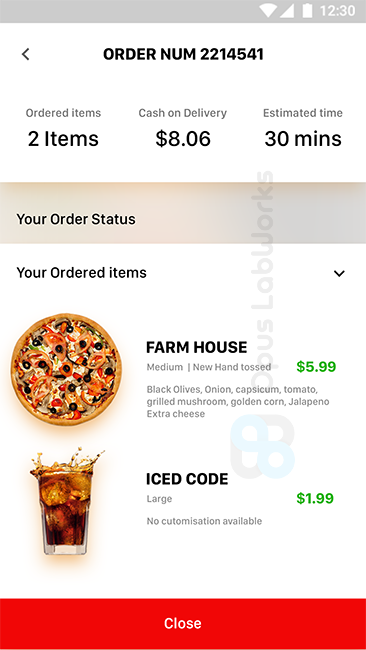This image, captured on a mobile phone, displays a detailed order summary from a food delivery app. At the top of the screen, a gray bar shows essential device information such as service signal, Wi-Fi status, battery level, and the time, which is 12:30 PM. These indicators, all in white, are located in the upper right corner. The page itself features a white background with the text "Order Number 221-4541" prominently displayed in the center. To the left of this text is a left-facing arrow icon, likely indicating a back navigation option.

Below the order number, the screen specifies the order details: "Ordered Items: Two Items," with the payment method listed as "Cash on Delivery: $8.06" and an estimated delivery time of 30 minutes. 

Following this information is another gray bar labeled "Your Order Status." Directly beneath this, a drop-down menu item titled "Your Ordered Items" is expanded, displaying the specifics of the items ordered. The first item is a "Farmhouse Pizza," medium-sized with a new hand-tossed crust. The toppings include black olives, onions, capsicum, tomato, grilled mushroom, golden corn, jalapeno, and extra cheese, all for $5.99. The second item is a large "Iced Coke," priced at $1.99, with no available customization options.

At the bottom of the screen, a red bar contains the word "Close" in white lettering, providing an option to exit the order summary menu.